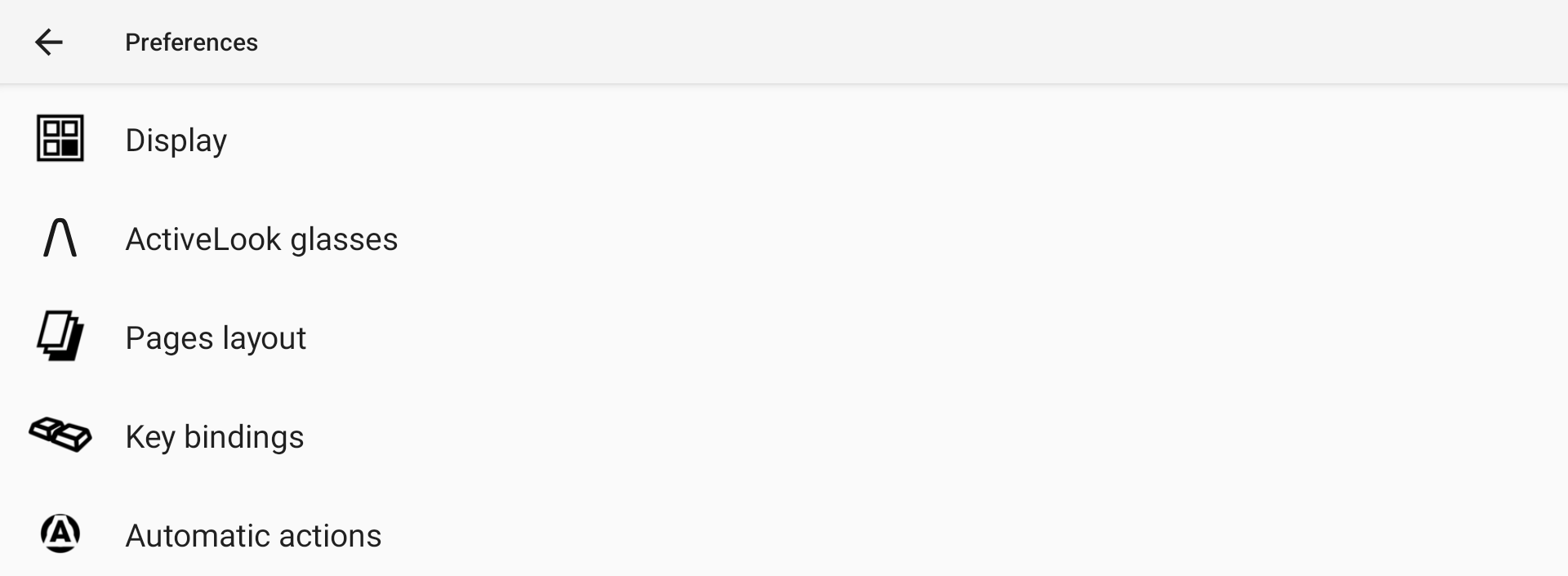This rectangular image features a user interface layout with the long side extending horizontally from left to right. The upper section of the image has a very light gray border, followed by an even lighter gray section below it. At the top left corner, there is a black arrow pointing to the left, accompanying the text "Preferences." 

Underneath, a series of black icons with accompanying labels are displayed. The "Display" icon, which is a square within a square, features four small squares inside it, with one of the squares filled in black. An upside-down 'V' icon is labeled "Active Look Glasses" and appears next to a depiction of several pages stacked together with the label "Pages Layout."

Additionally, there is an icon of two keyboard keys side by side, labeled "Key Bindings." Lastly, a black circle containing a white, highlighted letter 'A' is labeled "Automatic Actions." The entire interface design is in black on a light gray background and these are the only elements present in the image.